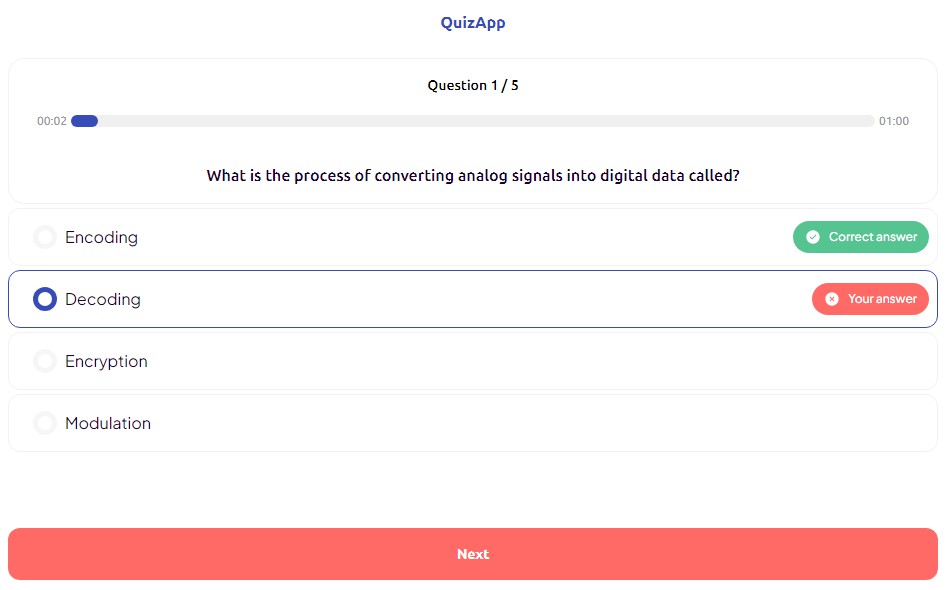The image depicts a screenshot of a quiz app interface set against a white background. At the top, in blue text, it reads "Quiz App", followed by a thin dividing line. Below this, the text "Question 1 of 5" is displayed. Underneath, a more prominent blue progress bar indicates the user's current position within the quiz. The question presented asks, "What is the process of converting analog signals into digital data called?" 

Four answer options are provided, each with a circular radio button for selection: 
1. Encoding 
2. Decoding 
3. Encryption 
4. Modulation 

The option "Decoding" is circled, indicating it was selected by the user, and is highlighted with a blue square around it. A red text underneath the selected option reads "Your Answer," while a green button above it displays "Correct Answer." The correct answer, "Encoding," is presumably marked within this indication. Below the answer options, there is a large pink button labeled "Next" for progressing to the next question.